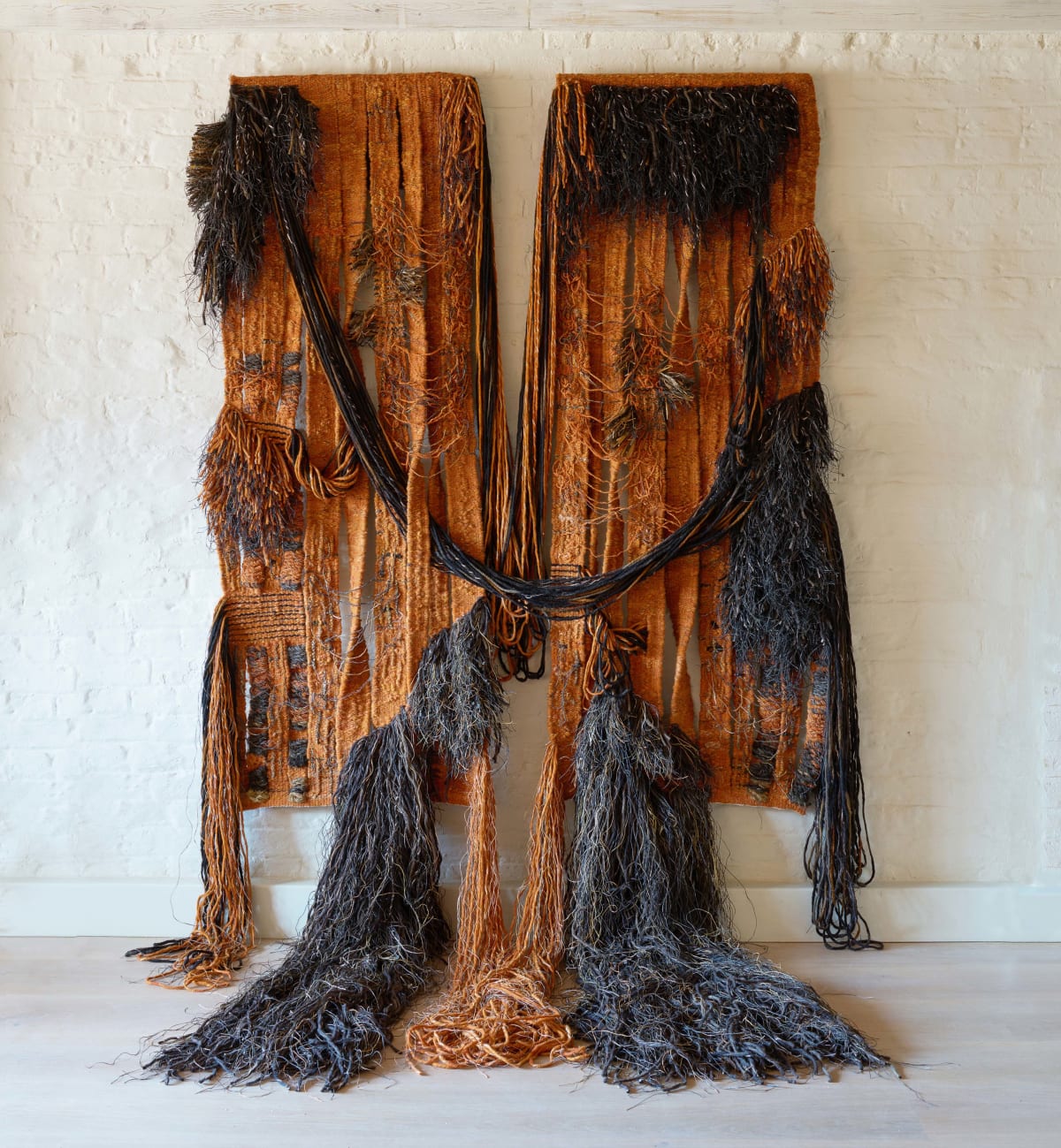This vertically aligned rectangular image, taken from a standing position, captures an indoor setting featuring a light-colored natural wood or stone floor at the bottom. Above the floor, a white baseboard transitions into a beige or off-white painted brick wall. Dominating the middle and upper portion of the wall is a hanging decoration consisting of two vertically aligned rectangular pieces arranged side-by-side. These pieces appear to be ornate and could be interpreted as curtains, rugs, or woven wall hangings. They are primarily orange with varying shades of brown, light brown, and rust tones.

Each rectangle is adorned with shaggy brown and medium-brown fabric or rope, creating a textured and somewhat shredded appearance. At the top, a thick, black rope interlaces from the left piece, arches down between the two, and connects to the right piece, further embellished with intertwining strips of rope. The bottom edges of these rectangles feature black tassels that resemble hanging hair, interspersed with occasional brown strands. Some of these shaggy elements extend all the way to the floor, adding to the intricate and tactile quality of the display.